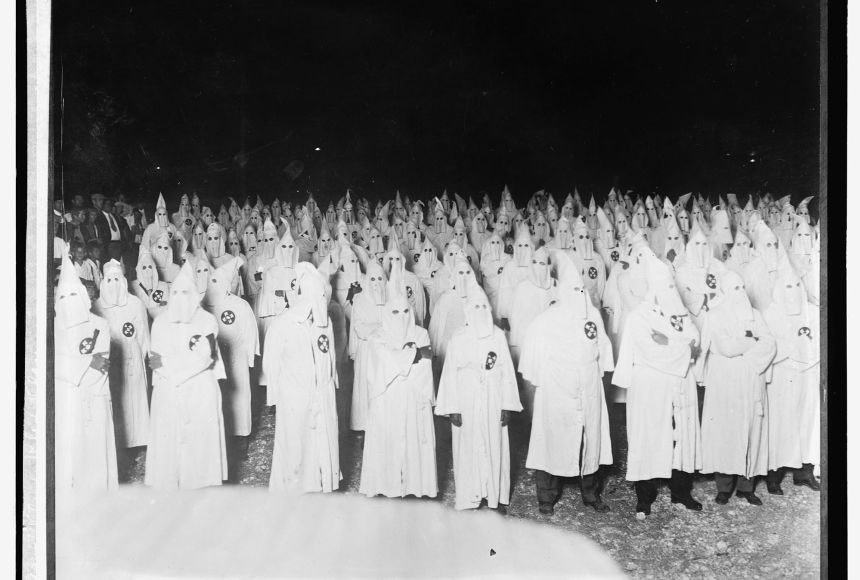The black and white photograph depicts a large, organized crowd of Ku Klux Klan members standing outdoors on what appears to be grass, under a dark nighttime sky. The Klan members are uniformly dressed in their iconic long white robes and pointed hoods with eye holes, resembling ghostly figures. Each robe features a distinctive emblem on the upper right chest area, described as a white cross or star-like symbol on a black circular background. The image shows lines of these hooded figures on either side, with black and white stripes from shadows or lighting effects adding to the atmospheric scene.

In the background, there are spectators dressed in regular attire, including suits, ties, and some white shirts, observing the Klan members. These onlookers include men, women, and children, adding an eerie contrast to the scene. The lower left part of the photo displays a mysterious white circular object on the ground, further contributing to the unsettling atmosphere of the gathering.